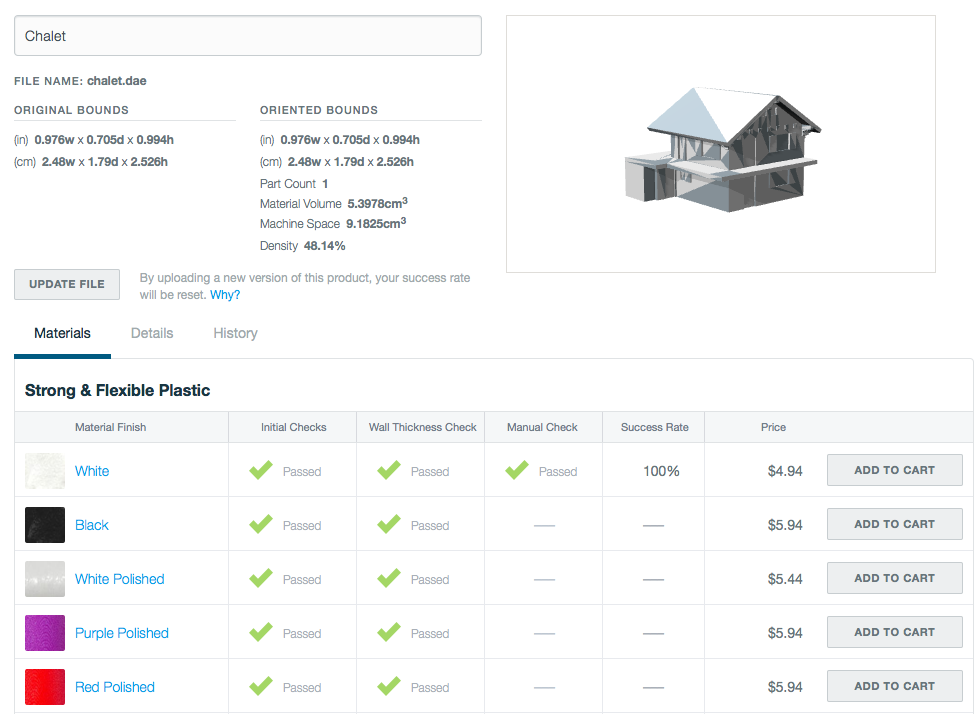**Detailed Image Description:**

The image displays a detailed summary of a file on a webpage or software interface. 

In the upper left corner, there is a search bar with the term "CHELIT" entered. Directly below this, in uppercase letters, is the label "FILE NAME:" followed by the file name "chelit.dae." 

The dimensions of the file are presented in two side-by-side tables that compare the original bounds to the oriented bounds. The original bounds are specified in inches as 0.976 W x 0.705 D x 0.994 H, with the equivalents in centimeters being 2.48 W x 1.79 D x 2.526 H. The oriented bounds are identical in measurement to the original bounds, both in inches and centimeters. 

Additional information is provided below these tables, including:
- Part Count: 1
- Material Volume: 5.3978 cm³
- Machine Space: 9.1825 cm³
- Density: 48.14%

To the right of the bounds tables, there is a rectangular section with a gray border and white background showing a digitally rendered image of "CHELIT." The illustration resembles a house with a roof divided diagonally into two colored triangles: a blue one on the bottom left and a white one on the top right. The rest of the house is shaded in various grays, from a tannish light grey to a darker bluish grey.

Toward the middle of the page, there's an action button labeled "Update File" in darker gray text on a gray background, accompanied by a clickable "Y link." 

Beneath this section, three tabs are available for selection: "Materials," which is currently selected as indicated by a blue underline, "Details," and "History." 

In the "Materials" tab, bold headline text reads "Strong and Flexible Plastic," followed by a table summarizing different plastic finishes. The table has multiple columns:
- Material Finish
- Initial Checks
- Wall Thickness
- Manual Check
- Success Rate
- Price

The price column, the rightmost, lists prices alongside gray "Add to Cart" action buttons. The table contains five rows with the following prices from top to bottom: $4.94, $5.94, $5.44, $5.94, and $5.94. The first row, which is the only one with a 100% success rate, features a green check mark under the manual check column and is labeled "White." All rows have passed the initial checks and wall thickness, indicated by green check marks.

The material finishes are shown with examples and names in blue fonts. The finishes include:
- White
- Black
- White Polished
- Purple Polished
- Red Polished